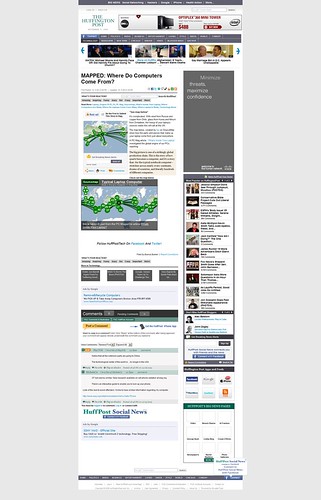This image captures a detailed view of the Huffington Post website, displayed in a particularly elongated format which allows for a broad, yet somewhat difficult-to-read, perspective of the entire page. At the top, the recognizable "Huffington Post" logo is visible in its signature green, establishing the site as a reputable news outlet. The primary focus of the page is an article titled "Mapped: Where Do Computers Come From?" A prominent graphic accompanies this article, illustrating a central point with green lines radiating to various locations, likely indicating the origins of computer components.

To the right, there is a gray sidebar featuring an advertisement, though the specifics of the ad are unreadable. Further down, another section displays a series of approximately eight images, each with corresponding text that appears to describe different articles. These smaller images and text snippets provide visual teasers for other content available on the site.

At the top of the page, additional links for various articles and ads are present, offering more content for users to explore. The bottom section of the page features the "HuffPost Social News" link, including an option to connect or log in via Facebook, thereby integrating social media interactions. Overall, the website showcases a variety of articles, with "Mapped: Where Do Computers Come From?" being the highlighted feature.